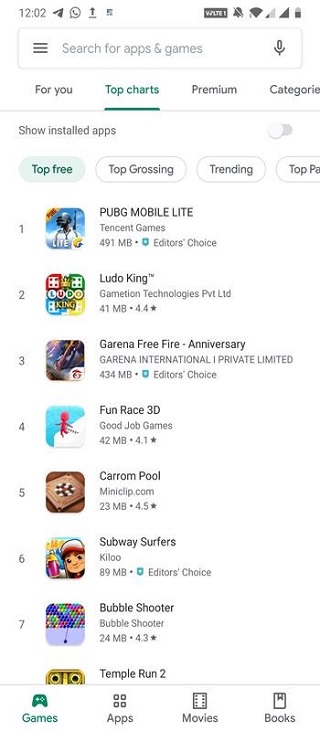Screenshot of the Google Play Store on a smartphone:

The image displays a screenshot from the Google Play Store with a predominantly white background. 

**Status Bar:**
- The top status bar includes several icons:
  - **Top left corner:** The time is displayed.
  - Following this, there is a series of icons:
    - An arrow icon.
    - A phone icon.
    - A download icon.
    - An indiscernible icon.
  - **Top right corner:** 
    - A battery icon showing half charge.
    - A signal icon with full bars.
    - Another signal icon with one out of four bars.
    - A full Wi-Fi icon.
    - Notifications are turned off.
    - A black rectangle with "VOLTE" inscribed in white.

**Search Bar:**
- Directly beneath the status bar, a search bar spans the width of the screen:
  - **Left side:** Three horizontal black lines.
  - Beside these lines, the placeholder text says "Search for apps and games."
  - **Right side:** A microphone icon.

**Navigation Tabs:**
- Below the search bar, there are navigation tabs:
  - **Left side:** In black text, "For you."
  - Next to it, "Top charts" is written in green with an underline.
  - Further to the right, in black text, "Premium."
  - Following that, "Categories."

**Settings Toggle:**
- Below the navigation tabs:
  - **Left side:** "Show installed apps" in black text.
  - **Right side:** A toggle button set to off.

**Category Tabs:**
- A light blue background tab indicating categories:
  - In green, "Top free."
  - Adjacent to it, three white tabs with grey borders and text:
    - "Top grossing"
    - "Trending"
    - "Top PA" (partially cut-off, off the screen).

**List of Games:**
- Below the category tabs, a numbered list of games from 1 to 7:
  - Each entry includes:
    - A thumbnail image of the game.
    - The game’s name next to the thumbnail.
    - The game developer's name underneath.
    - The file size in megabytes.
  
**Bottom Navigation Bar:**
- Only the top half of an eighth game listing is visible at the bottom.
- Bottom navigation bar icons:
  - **Left to right:**
    - A green controller icon labeled "Games."
    - A black apps icon labeled "Apps."
    - A black movies icon labeled "Movies."
    - A black books icon labeled "Books."

This detailed description encapsulates all visual elements from the Google Play Store screenshot on a smartphone, providing clarity on the layout and content displayed.